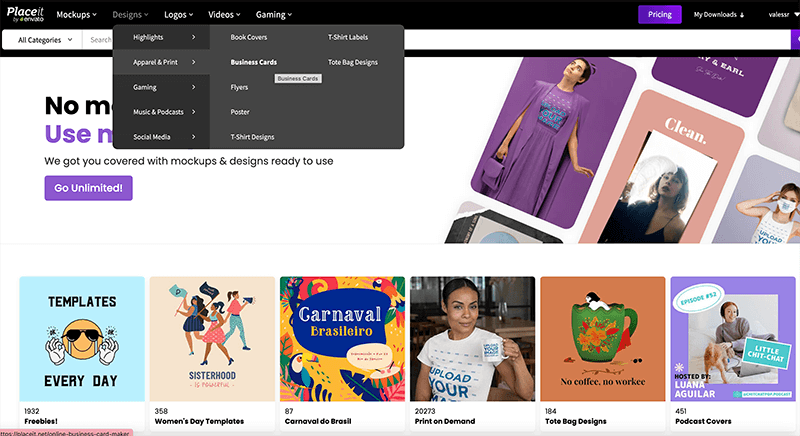This is a detailed screenshot of a web page belonging to the company "Placeit." The header at the top is black, featuring the company name "Placeit" in the left corner. The word "Placeit" is written in white font, with "Place" in bold and "it" in regular font, slightly lighter but still white. Beneath the company name, there is an additional word that is unfortunately too small to read.

The header also contains a top menu with categories: Mockups, Designs, Logos, Videos, Gaming. One of these menu items has a drop-down menu visible, which appears as a dark grey box. This drop-down menu features sections titled: Highlights, Apparel and Print, Gaming, Music and Podcasts, and Social Media. To the right, it lists specific items such as Book Covers, T-Shirt Labels, Business Cards, Tote Bag Designs, Flyers, Posters, and T-Shirt Designs.

The main content area of the web page, beneath the header, has a white background. This drop-down menu overlaps part of the main headline, allowing only a partial view of the text: "no M" in black and "use N" in purple. Below this, in grey font, it reads, "We got you covered with mock-ups and designs ready to use." There is a purple rectangular button with white text that says "Go Unlimited."

At the bottom of the page and on the right side, there are various examples of the types of designs available. Categories include Freebies, Women's Day Templates, Carnival Brazil, Print on Demand, Tote Bag Designs, and Podcast Covers. Each category is illustrated with example photos. For instance, under Print on Demand, there is a photo of a medium to dark-skinned Latina woman wearing a white t-shirt that partially reads, "Upload your," with the rest of the text not visible. These visuals showcase the range of customizable design templates that Placeit offers, highlighting its print-on-demand service.